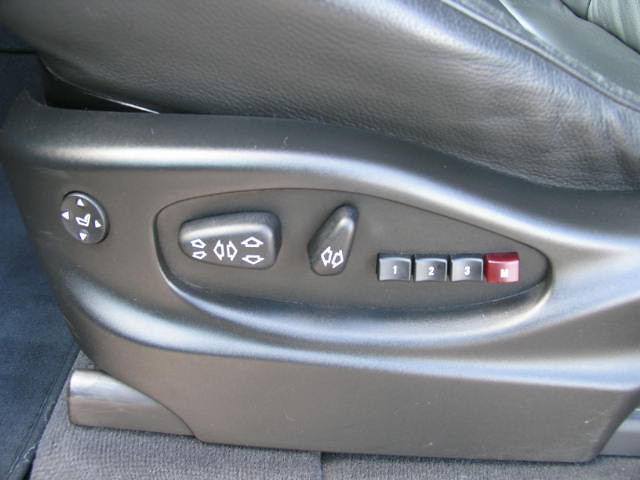The image showcases a close-up of the controls for a gray leather car seat, which rests on a metallic base with a silver finish on a gray surface. The buttons are housed in a recessed, oval-shaped segment of the seat's side, made primarily of a stiff plastic or silvery gray material. The central part of this control panel features a circular button with arrows pointing in all four cardinal directions, indicating multi-directional seat adjustment capabilities. Adjacent to this circular button is a wider rectangular button with vertical and diagonal arrows, and a smaller oval (or egg-shaped) button below it, marked with horizontal arrows. Further to the right, there are three grey buttons labeled "1", "2", "3", and a larger bright red button that either says "Pause" or has an "M" on it. The seat controls illustrate a modern, sleek design with the buttons providing various adjustment functions.